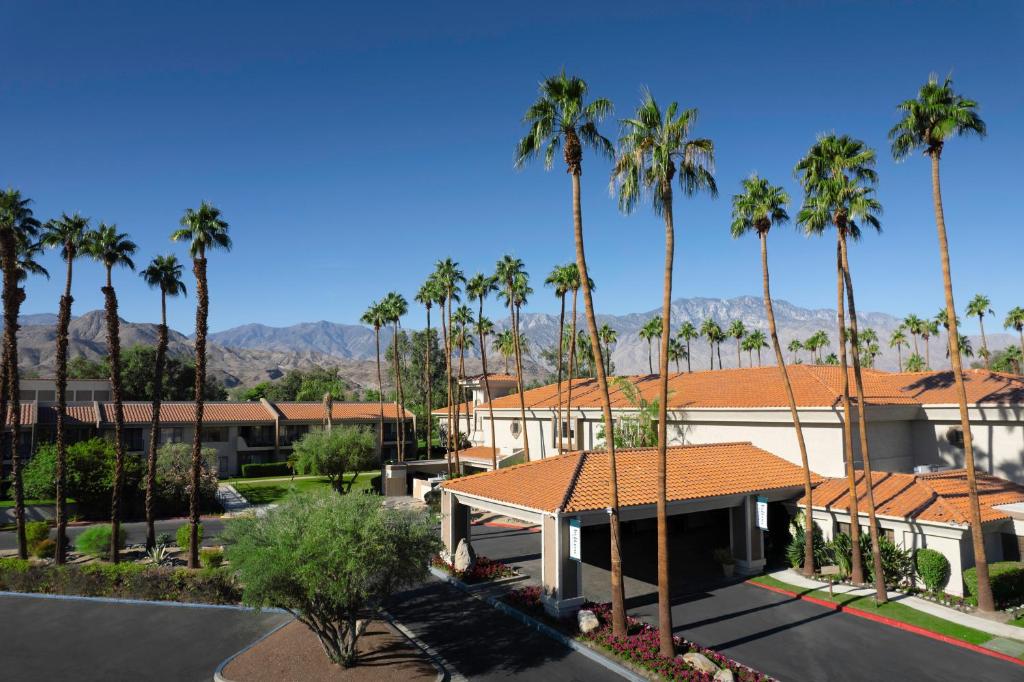This photograph captures an elevated, daytime view of the Hyatt Vacation Club at Desert Oasis, an upscale resort situated in Palm Springs, California. Dominating the scene are three main buildings adorned with adobe-colored shingle roofs and framed by numerous tall, slender palm trees, distinctive for their elongated trunks and delineated fronds. The central building, which features a canopy over the driveway, serves as the main entrance, welcoming guests as they arrive. To the left, a long building extends towards the photograph's edge, while a smaller structure is positioned just right of the canopy.

In the foreground, a neatly landscaped area with hedges, shrubs, and other greenery borders a driveway that connects to a parking lot on the photo's lower left-hand corner. The resort's lush vegetation contrasts beautifully with the stark, gray-brown mountains in the background, emphasizing the desert locale. The mountain range, though slightly hazy, sets a dramatic backdrop, spanning the midline of the rectangular image. Overhead, the clear blue sky deepens in shade as it ascends, creating a stunning gradient from light blue near the horizon to a rich azure at the top. This meticulously designed resort, nestled in a classic California desert landscape, exudes luxury and tranquility, epitomized by its serene ambiance and the natural beauty surrounding it.